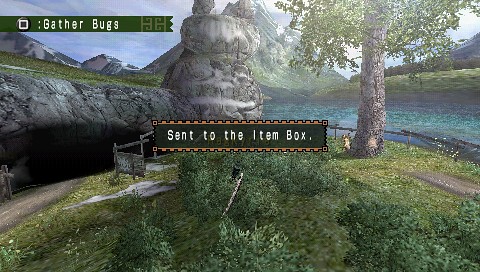This is a color screenshot from an older video game, characterized by its dated graphics. The image showcases a lush, grassy area filled with various green foliage and plants, predominantly in the bottom half of the image. To the right, there's a prominent tree with numerous leaves, and behind it, a stream of water extends towards the background where a mountainous region looms large. In the top left corner, a dark cave or alcove is visible, partially obscured by some stone columns.

Two distinct in-game interface elements are notable: at the top left, set against a green ribbon, is the text "gather bugs," accompanied by a black circle with a white square inside it. Centrally located in the image is a white caption that reads, "sent to the item box," indicating that an item, likely a bug, has been collected and stored. The overall composition of the image is wide, capturing a serene and naturalistic environment with no presence of people, animals, buildings, or signs.